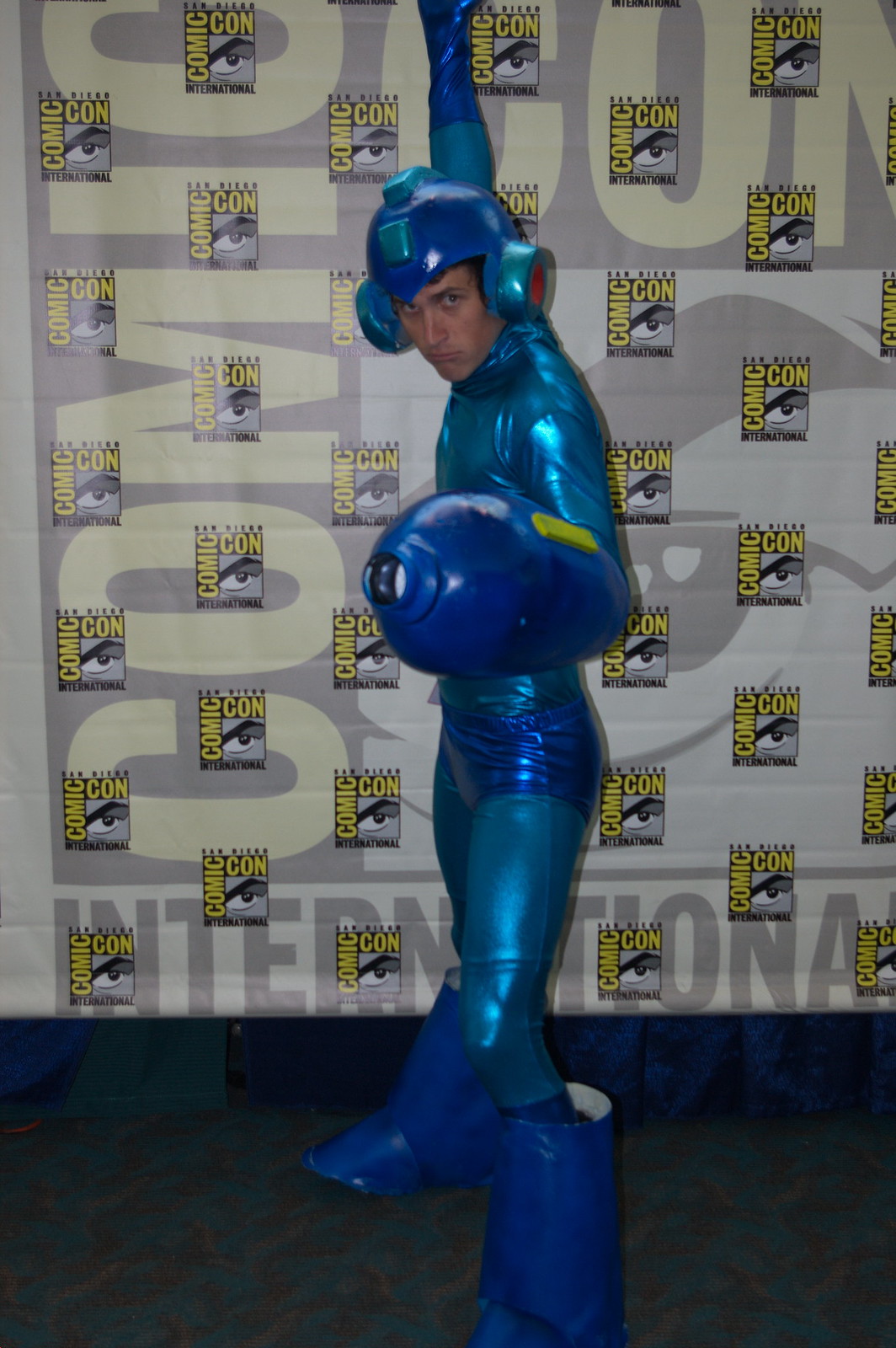This is a vibrant vertical color photo taken at Comic-Con, featuring a young man in an incredibly detailed Mega Man cosplay. The man is standing on a blue carpet in front of a backdrop adorned with numerous Comic-Con logos and the words "Comic-Con International." His costume is a shiny, rubbery, medium blue bodysuit, complemented by darker blue shorts and sizeable coordinating blue boots. His blue helmet has distinct red and blue blinker-like features on it, and you can glimpse a bit of his dark hair peeking out. The man’s right arm is raised, adorned with a blue glove, while his left arm is encased in a large, blue, tank-like blaster that resembles an oxygen tank. He’s captured in a dynamic pose, seemingly ready to "blast" as he looks directly at the camera, exuding the classic Mega Man spirit. The backdrop and the detailed precision of his attire confirm that he’s among the enthusiastic cosplayers showcasing their impressive costumes at this bustling Comic-Con event.